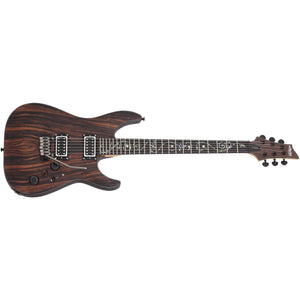This detailed photo features an electric guitar set against a completely white background. The guitar showcases a rich, multi-colored wooden body with varying grains in light brown, dark brown, and black, creating a visually striking, marbled appearance. The instrument is oriented sideways in the image and appears to be positioned upside down, revealing its intricate details. 

The left side of the guitar, viewed from this orientation, includes a black knob and a gray whammy bar, along with the beginning of a black fretboard edged in gray. The fretboard contains a series of white dots marking the frets. At the top end of the neck, six metal tuning knobs are arranged, three on the top and three on the bottom. 

The guitar strings, also visible, are attached at both ends, with their base connecting to metallic components. Although primarily adorned in brown and black hues, there are subtle hints of blue among the strings. The overall design and features clearly indicate that this is an electric guitar without any accompanying text or additional elements in the image.